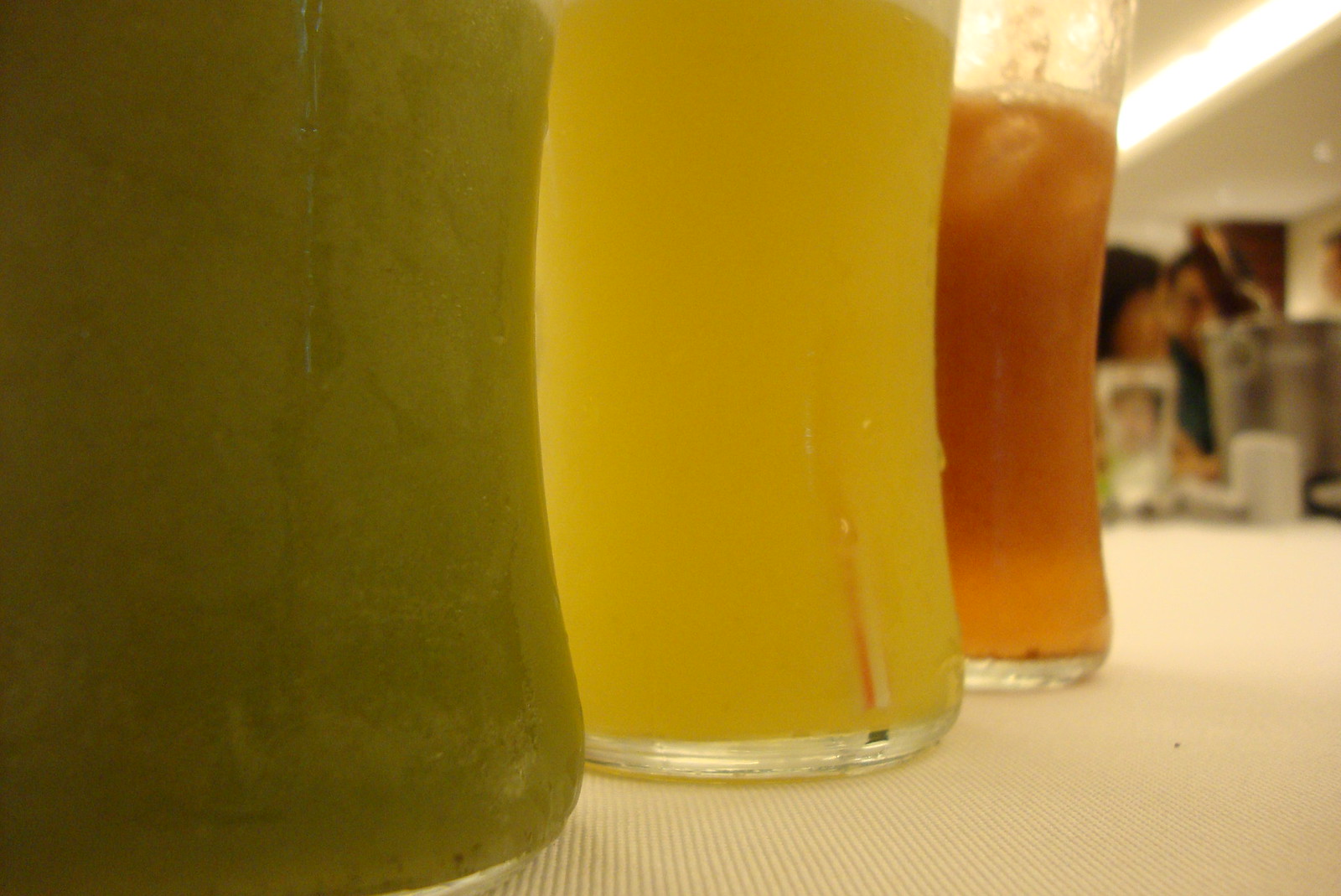The image captures an extreme close-up of three clear, tall glasses displaying different beverages, situated on a textured beige surface that is likely a table with a white tablecloth that has some knitting. The focus on these glasses is so tight that only the bottoms are visible. Each glass contains a distinct liquid: the one to the left contains an olive green drink, possibly a kale smoothie or a kiwi-flavored beverage. The middle glass holds a yellowish liquid, which could be lemonade or a light pineapple juice, given its translucent, thin appearance. The rightmost glass has a brownish-red liquid that might be iced tea or a blood orange cocktail, with evidence that someone has taken a sip.

All three glasses exhibit condensation, indicating they are cold. In the blurred background, which features a white wall and ceiling, there are a few people seated at the table. One person, possibly with dark hair and of Asian descent, seems to be holding a bucket-like object. Additionally, a rectangular, warm glowing light can be seen on the upper right side of the photo, contributing to the overall warm, colorful ambiance of the scene.